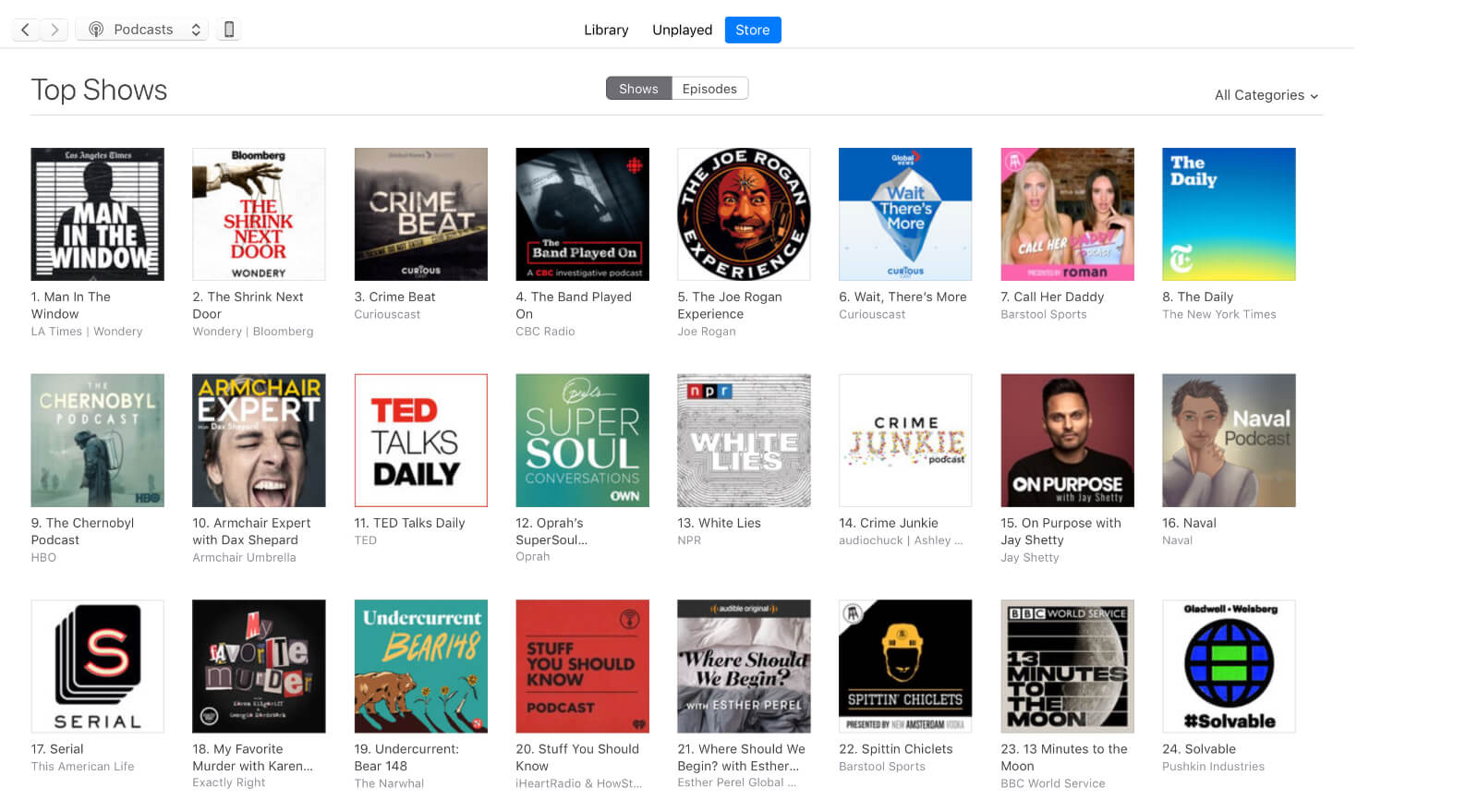This image depicts a digital podcast interface set against a white background, featuring various navigational aids and elements. At the top, there are left and right arrows along with an icon representing a podcast with up and down arrows. Below, there are three main tabs labeled "Library," "Unplayed," and "Store." The "Store" tab is highlighted with a blue rectangle, while the "Episodes" section is underscored with a gray rectangle. A further white rectangle introduces the section "Top Shows in All Categories," which lists several podcasts in a ranked order.

1. **Man in the Window** is listed as the number one podcast.
2. **The Shrink Next Door** appears at both the first and second positions.
3. **Krombeat** is ranked third.
4. **The Band Played On** is fourth, accompanied by an image of a shadowy man, suggesting a theme of spying or secrecy.
5. **The Joe Rogan Experience** holds the fifth spot, showing a man with a tattoo on his forehead.
6. **Wait, There's More** is sixth on the list.
7. **Call Her Daddy** is seventh and features an image of two women.
8. **The Daily** is listed eighth and repeated.
9. **The Chimbrel Podcast** (C-H-E-R-N-O-B-Y-L) is ninth, depicting a man who appears to have something on his back, possibly spraying.

This detailed description captures the visual and textual elements of the podcast interface.